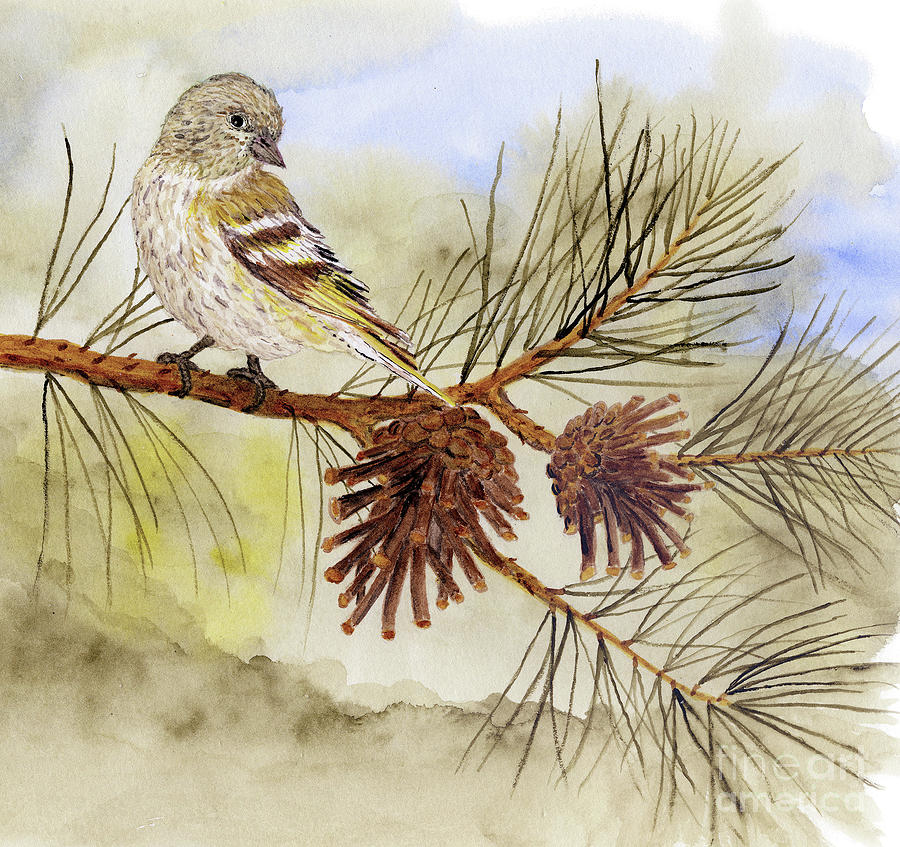The image depicts a watercolor painting of a bird perching on a sparse pine tree branch. The bird, perched on the top left, has a distinctive grayish-brown, feathery head, a tiny brown beak, and a light-colored belly. Its wings display a striped pattern of yellow, white, and brown, and the tail feathers are prominently yellow. The branch, emanating from the left, splits into three smaller branches adorned with thin, sparse pine needles, making the needles easily visible. At the base of the branch are two spiky pine cones, whose hard segments are closely packed together at the bottom and more spread out towards the tips. The background consists of a watercolor wash, combining hues of gray, yellow, and blue that evoke a cloudy, foggy day. At the bottom of the painting, a watermark reads "Fine Art America."